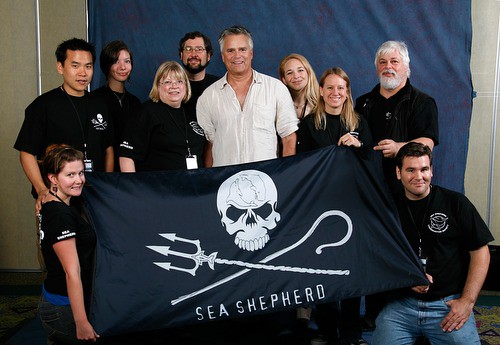In the image, a group of men and women, both young and old, is gathered in front of a blue backdrop. They are posing together, most of them smiling, with two people kneeling in the front. The woman on the left and the man on the right are both wearing black shirts and blue jeans, though his jeans are lighter than hers. The man has black hair. Most of the group members are dressed in black t-shirts, while the man standing in the center behind a banner is noticeable in a white button-down shirt with rolled-up sleeves. He has dark and silver hair. The banner they hold is black and displays a white skull with dolphins on its forehead, crossed by a trident and a staff underneath it, with the words "Sea Shepherd" written below. Although the exact attire of everyone is not entirely clear, the message and the unity of the group are prominently conveyed by their smiles and coordinated appearance.